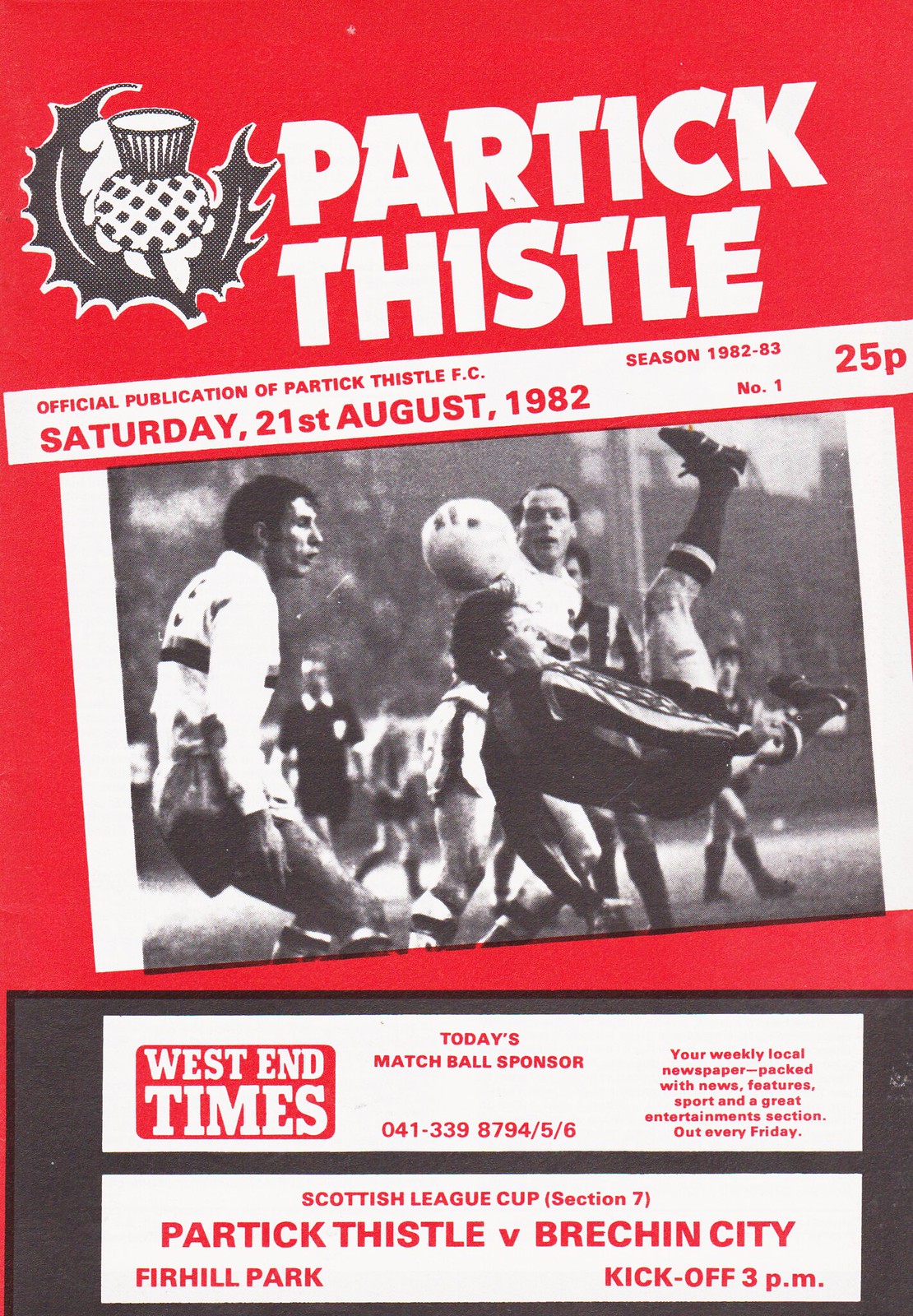The image is a program cover for a football match featuring a striking red background with prominent white lettering reading "Partick Thistle" at the top, accompanied by a thistle emblem in the top left corner. Below, it is titled "Official Publication of Partick Thistle FC Football Club, Season 1982-83," with additional details: "Saturday, 21st August 1982, Number one, 25p" on the right. The central feature is a black-and-white photograph of soccer players in action, with one player airborne mid-kick amidst several others. Beneath the angled image are two advertisement panels, one specifying "West End Times, Today's Matchball Sponsor," and further text inviting readers to their newspaper full of news, features, and entertainment. The bottom of the program announces the match details: "Scottish League Cup Section 7, Partick Thistle vs. Brechin City, Firhill Park, Kickoff, 3 p.m."